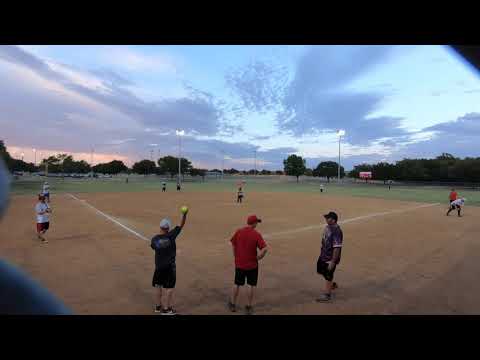An image of a likely softball game, taken through a hole in a fence, possibly with a fisheye lens. The dirt field is marked with worn white chalk lines, tracing from home plate to first and third bases, indicating heavy use. At the center, a man dressed in dark shorts and shirt, and a white hat, is holding a large yellow softball aloft, signaling a play. To his right, another man, wearing a red shirt, red hat, and black shorts, stands, possibly the umpire. A third man in a baseball cap approaches them. Along the first and third baselines and scattered in the infield and outfield, various players are positioned, ready for play. The field is predominantly dirt in the infield, transitioning to green grass in the far outfield. The absence of a batter suggests the game might be between innings.